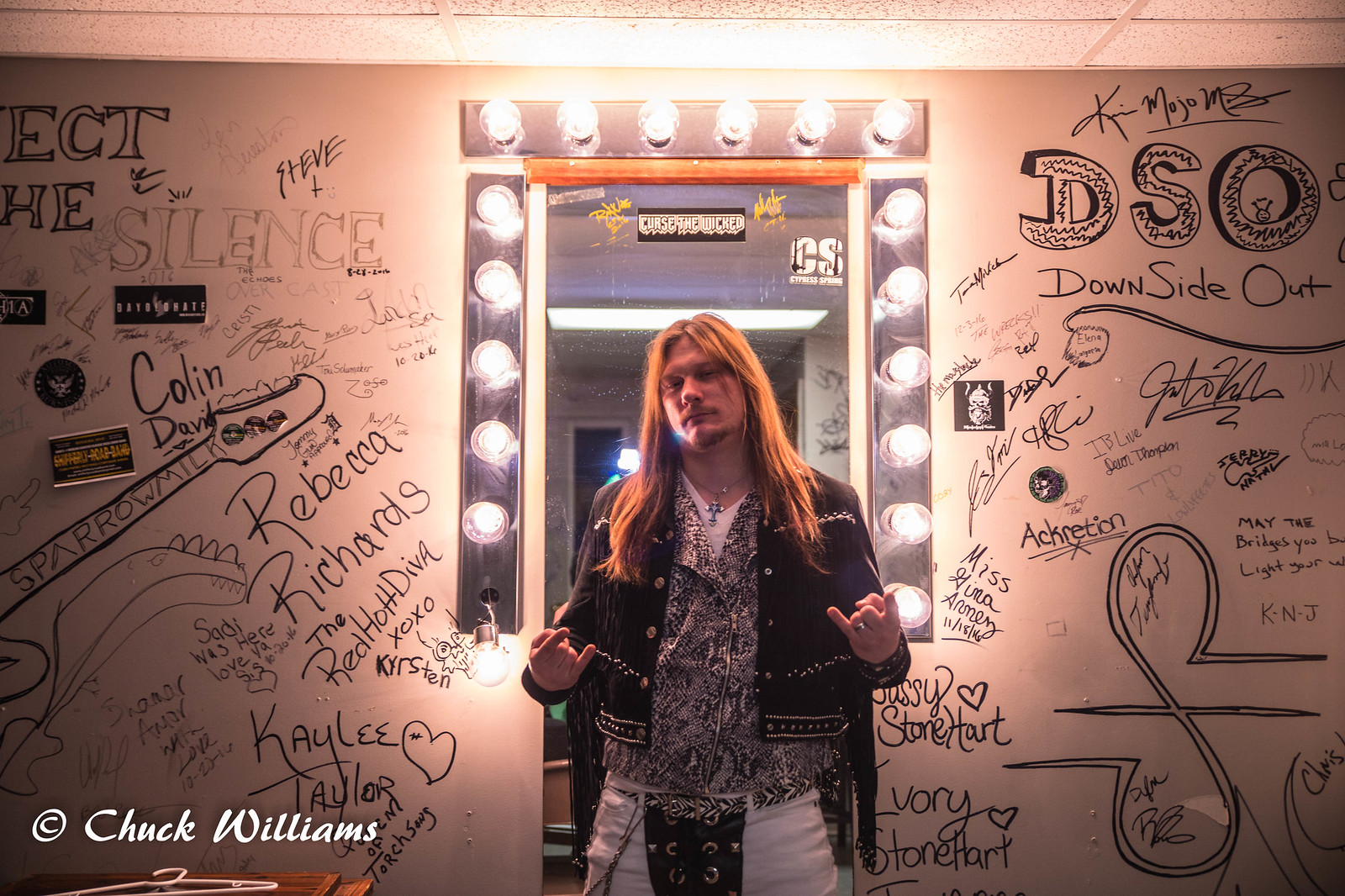The image features a man with long reddish-brown hair standing in front of a brightly lit makeup mirror, the type surrounded by numerous bulbs. He appears to be a rock performer, as evidenced by his "rock devil horn" hand gesture and his edgy attire—a black jacket with tassels, layered over a gray, black, and white jacket that zips up, and a white shirt underneath. He also wears a cross necklace and striking white pants adorned with a black background and silver eyelets, laced up across his lower area. The setting is a white wall covered with black signatures and graffiti, reminiscent of autographs from various people. In the lower left-hand corner of the image, the text "at Chuck Williams" or "Copyright Chuck Williams" suggests that the man might be Chuck Williams and indicates the photo might be taken in his dressing room or a similar personal space.